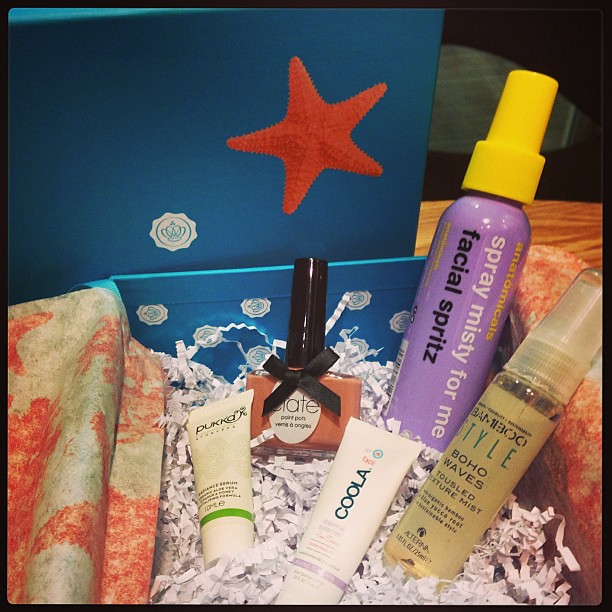This image captures an Instagram-worthy unboxing of a luxurious dark ocean blue gift box adorned with a red starfish and a small white circular logo featuring an illustration of a crown. The box, propped open on a wooden table, reveals an intricate pattern of small white logos lining its interior. The contents are nestled in shredded white crinkle paper and coral white gift paper. Inside, you'll find several beauty product samples, including a "Misty for Me" facial spritz in a purple and yellow bottle, a "Bamboo Style Boho Waves" tousle texture mist for hair, a brown nail polish with a black lid and bow, a white travel-sized tube of "Perka" lotion or cream, and another travel-sized tube from "Coolo" brand. The slightly brownish tissue paper with orange splotches adds a decorative touch, enhancing the aesthetic appeal of the carefully curated gift box.